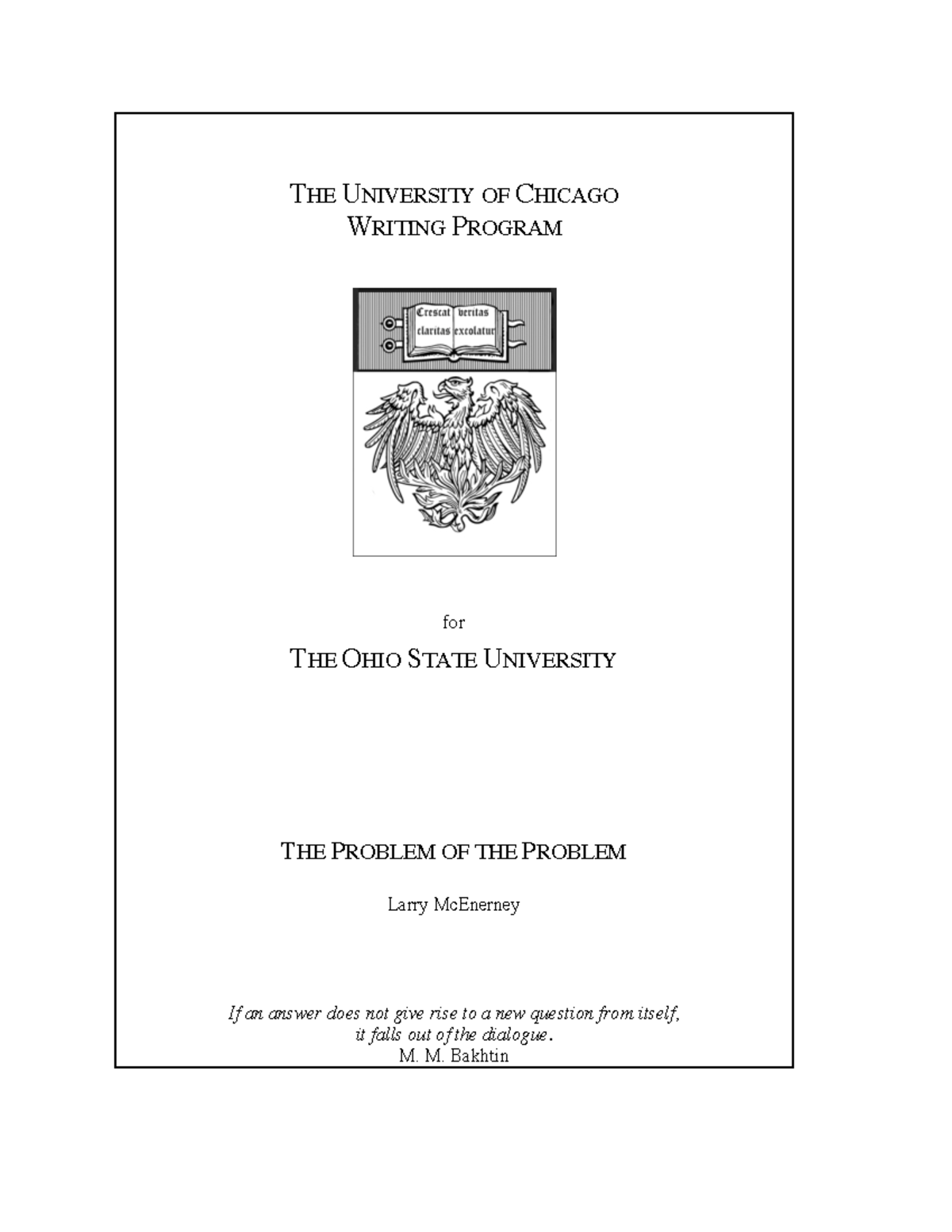The image features a clean, white background with a thin rectangular outline. At the top, in uppercase text, it reads "THE UNIVERSITY OF CHICAGO." Directly below this, also in uppercase, is the phrase "WRITING PROGRAM." Centrally positioned is an emblem depicting an open book, with visible white pages set against a gray background. Below the book, a large bird, resembling a phoenix, is illustrated with outstretched wings, rendered in shades of black and gray with detailed shading.

Further down, in smaller text, the word "FOR" (spelled out as F-O-R) is written. Beneath this, in bold and uppercase text, it reads "THE OHIO STATE UNIVERSITY." About three inches down from this, the text "THE PROBLEM OF THE PROBLEM" is displayed in bold, uppercase letters. Below this title, in smaller text, the name "Larry Montgomery" is mentioned with the quotation: "If an answer does not give rise to a new question from itself, it falls out of the dialogue." 

Finally, at the bottom of the image, in bold black text, the characters "M.M.B-A-K-H-T-I-N" are listed, marking the end of the text.